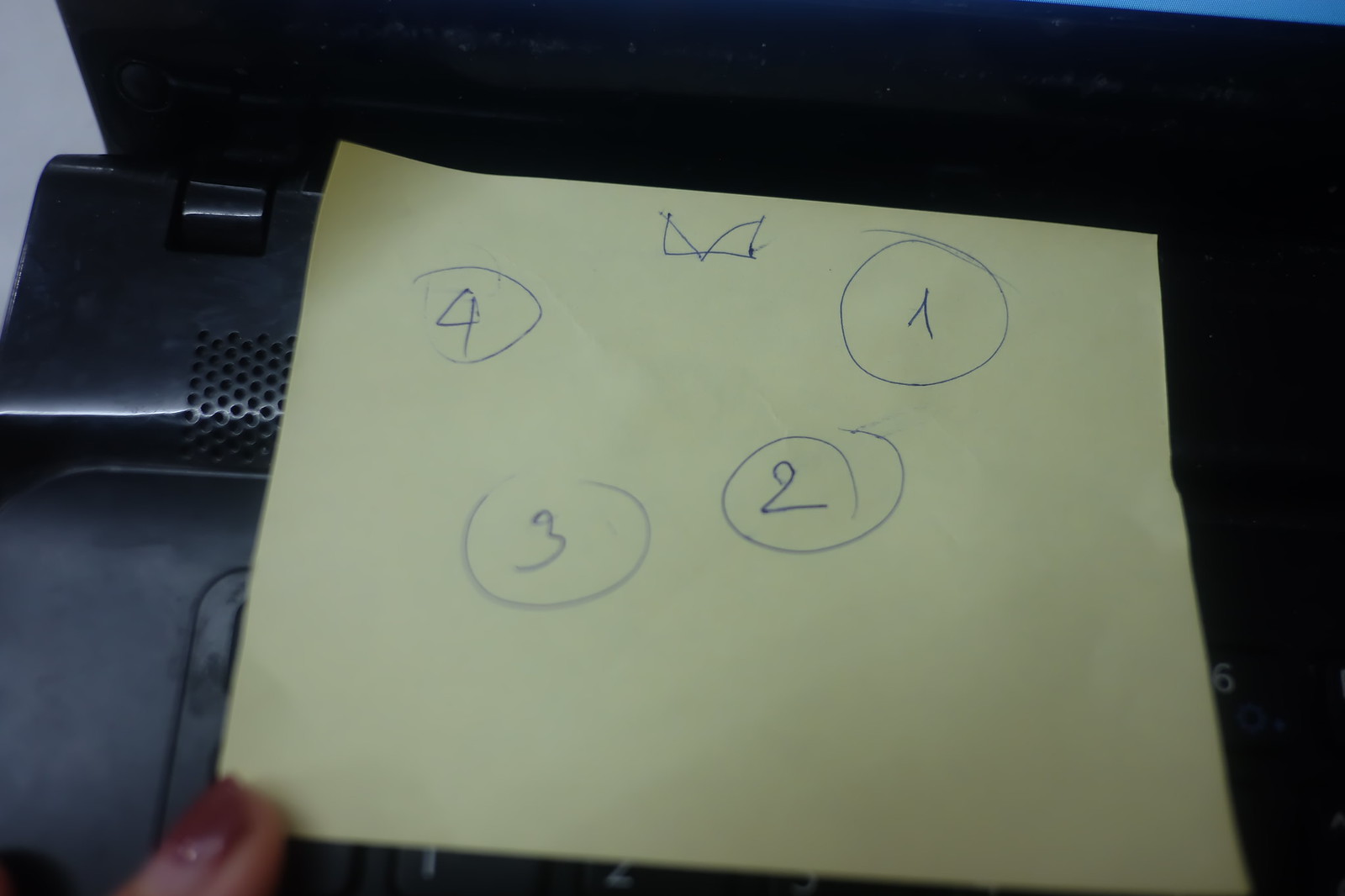In this image, an adhesive sticky note is affixed to the corner of a black computer, captured in a somewhat blurry, lower-quality photograph, likely taken with an older camera. The sticky note prominently features a series of four circles, each numbered sequentially from right to left as 1, 2, 3, and 4. Above the numbered circles, there is a drawing resembling two facing triangles, meeting at their vertices and forming a straight line at the bottom, resembling an "M" shape. The backdrop includes the upper left-hand corner of the computer's keyboard and a small portion of the screen at the top. In the lower-left corner of the photo, a person's finger with somewhat opaque, red nail polish is visible, partially obscuring the view.